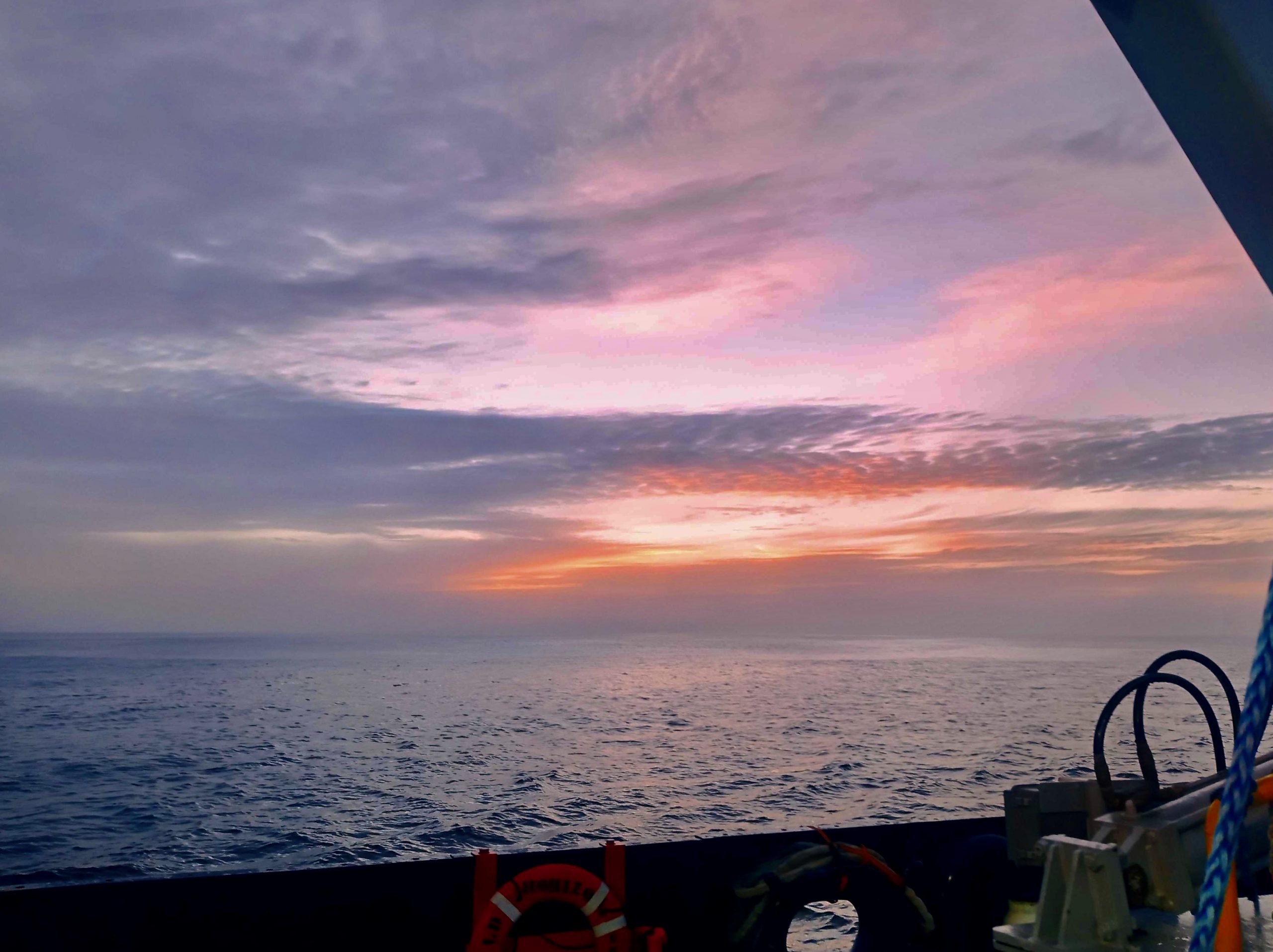This color photograph, taken from the deck of a boat, captures the serene beauty of either a sunrise or sunset over the ocean. The sun is nearly below the horizon, casting a glow of vibrant orange that transitions to pink as it ascends the frame, illuminating the cloud-filled sky. The horizon lies beneath a horizontal deck of grayish blue clouds, while higher up, the sky mingles with puffy white and gray clouds tinged with orange and pink.

The calm ocean waters near the boat are a deep crystal blue, gradually lightening to a teal or turquoise hue towards the horizon. In the lower foreground, an orange, round life preserver is prominently displayed, hanging on the interior side deck wall of the boat. Adjacent to it, in the bottom right corner, there's a table on the deck with what appears to be food and snacks, and a tote bag with upright handles. The scene is backlit by the striking glow of the nearly set (or risen) sun. Adding structural detail, a diagonal beam, possibly part of the boat’s bridge or a canopy cover, cuts across the upper right corner of the image.